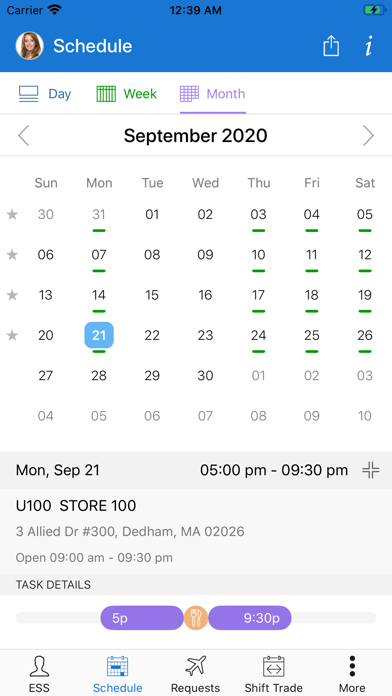The image is a screenshot of a cellphone displaying a detailed schedule. At the very top, there's a blue banner showing the carrier, the time "12:39 AM" in the center, and a green battery icon with a lightning bolt on the right. Next to a small profile picture of a woman with brown hair, the word "Schedule" is written just below the blue banner. The interface then transitions into a white background containing buttons for different view options: a blue button labeled "Day," a green button labeled "Week," and a purple button labeled "Month." The purple button has a purple line underneath it, indicating that it is currently selected.

The main portion of the screenshot displays a calendar for September 2020, with dates arranged from Sunday through Saturday. Several dates, specifically Monday, Thursday, Friday, and Saturday, are marked with green underlines, indicating events. The 21st of September is highlighted in blue, signifying a selected date.

Below the calendar, there's a detailed schedule entry for Monday, September 21, showing the event's time, location, and additional task details. The event is scheduled from 5:00 PM to 9:30 PM at "You 100 Store, 100 3 Alley Drive, Number 300, Dedham, MA 02026, open from 9:00 AM to 9:30 PM." Further details are provided in purple ovals, marking the times 5:00 PM and 9:30 PM.